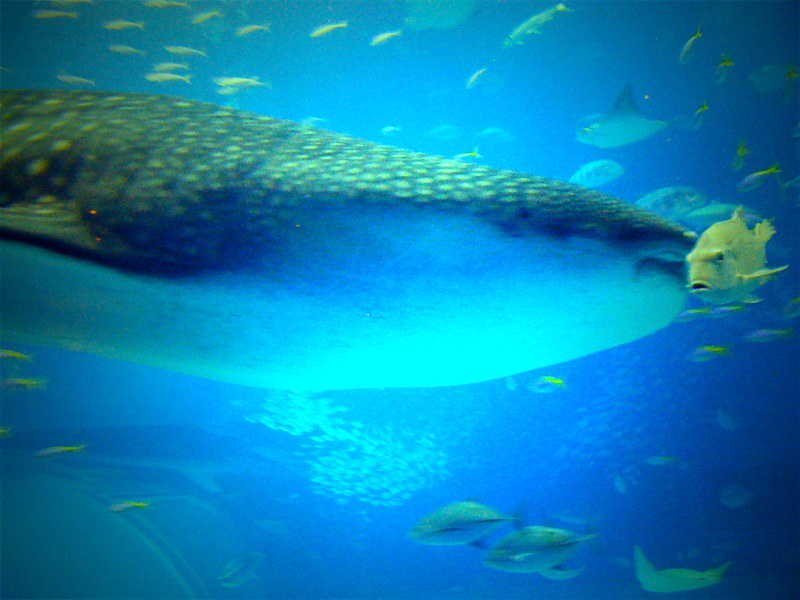The photograph captures the ethereal beauty of undersea life with a distinct blue natural filter typical of underwater images. Central to the composition is a large, tube-shaped fish, identifiable by its white underside and a gray back speckled with yellow spots. It has a tiny slit for a mouth, with small black eyes positioned on either side of its head. Adjacent to this prominent fish, a significantly smaller yellow fish with bulbous black eyes floats, seemingly unaffected by the presence of its larger companion. The top left corner of the image houses a minuscule completely yellow fish, adding to the variety of the aquatic scene. Scattered throughout the background are multiple other fish resembling the two central characters, contributing to the dynamic atmosphere. The photograph's corners are noticeably darker, imparting an old-timey feel, possibly enhanced by a filter effect. The overall out-of-focus presentation imbues the scene with a fuzzy, almost dream-like quality. The backdrop is populated with numerous smaller fish, primarily in shades of yellow, giving a sense of bustling underwater activity.